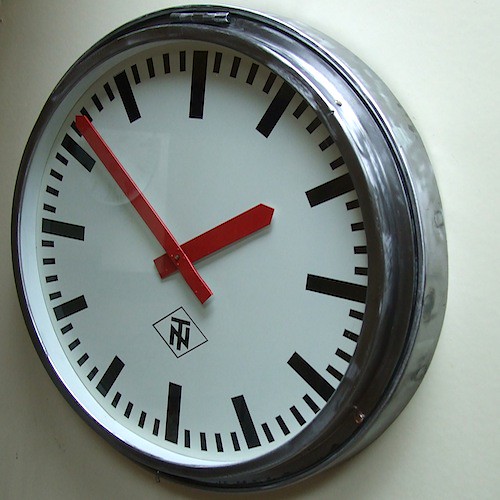This photo captures a round wall clock with a minimalist design, mounted on a white painted plaster wall. The clock features a face surrounded by a sleek stainless steel case, which is further encased by a larger, older, and slightly dinged metal frame. The clock face itself is white, devoid of numerals, and instead marked by thick black lines for the hours and thinner black lines for the minutes. Prominently, the clock's minute and hour hands are a vibrant cherry red, both thick and bold in appearance. Notably, above where the numeral 6 would typically be, there is a black square rotated to resemble a diamond, containing the initials "TN" in black ink. The glass of the clock face subtly reflects the image of another clock, just faintly visible in the background.